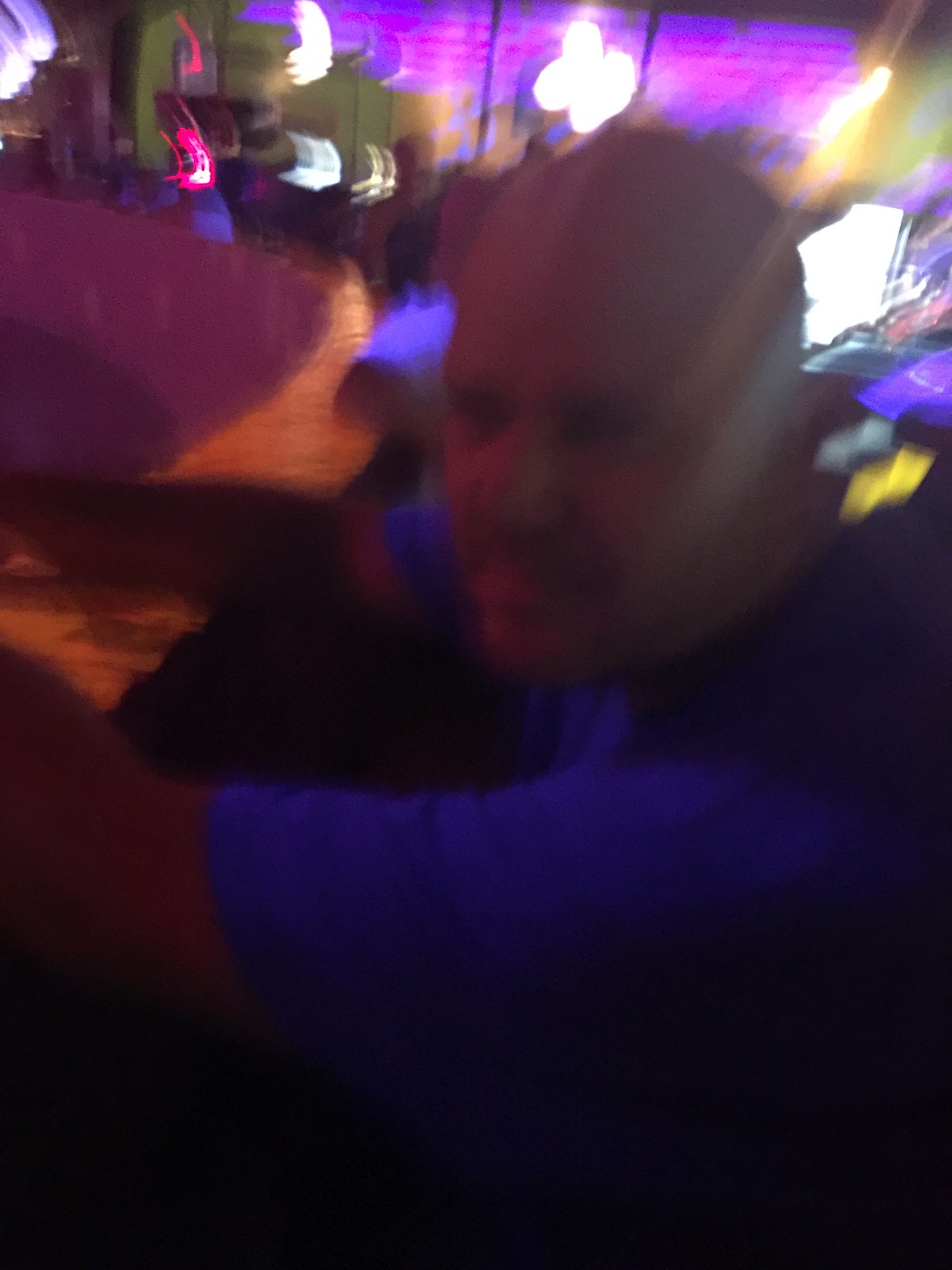In the extremely blurry and grainy photograph, a Hispanic man with brownish skin, dressed in a blue shirt, is captured in a side profile as he gazes towards the left. His head is shaved, and he sports a mustache. The man is slightly leaning forward, positioning his arms on a surface that appears to be either a stage or a bar, while seated lower than that surface. A noticeable purple blur is present on the stage, indicative of the camera's motion during the shot. The background reveals hanging lights from the ceiling, with illuminated machines that could be either arcade or slot machines adding ambient glow to the scene. A window is visible further back, obscured by a purplish distortion, contributing to the overall obscurity of the image.